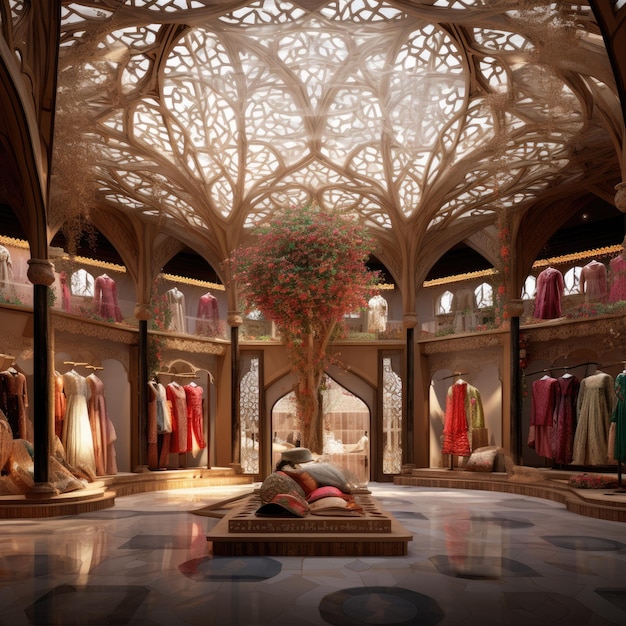The image is a full-color, vertically rectangular photograph of the interior of an upscale women's clothing store, with no border or text. The setting is clearly staged, emphasizing its high-end and unique aesthetic. The store's floor is made of glossy marble featuring decorative patterns in blues and browns, composed of circles and squares. The ceiling is designed to resemble bare tree branches, crafted in a tan color and interwoven to create a fantasy-like ambiance that allows sunlight to filter through.

Centrally located is a large tree growing in a low, rectangular planter box, adorned with green leaves and pink flowers. Surrounding this centerpiece are high-end women's dresses in various colors including white, red, burgundy, tan, and black, displayed on hangers and mannequins. The room's round shape is accentuated by black pillars extending upwards, supporting the intricate branch-like ceiling structure. The overall scene exudes a blend of natural elements and luxurious fashion, creating an enchanting shopping environment.